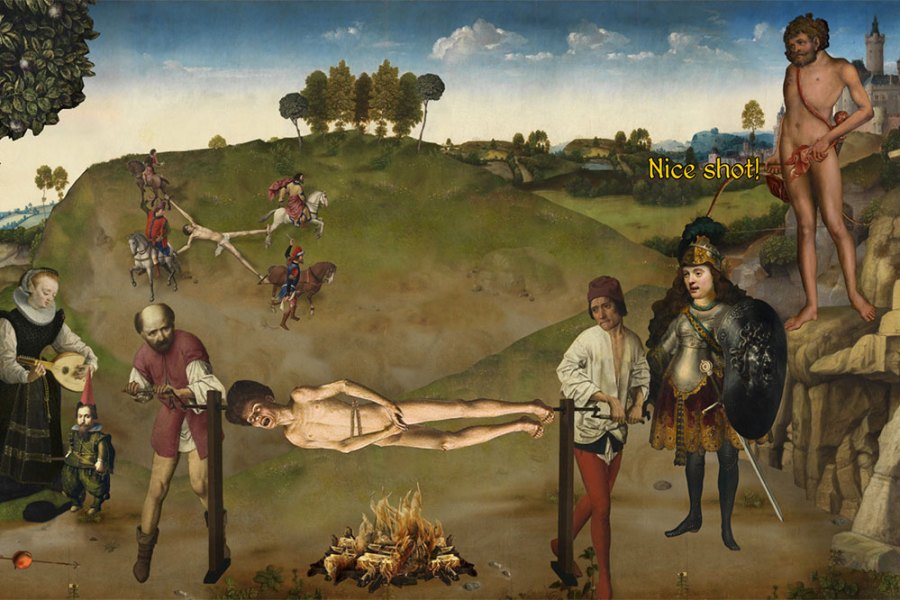The image is a highly disturbing vintage-style painting or colored drawing in a landscape layout. The top of the background features a bright blue sky filled with puffy white clouds, while the bottom is dominated by green rolling hills adorned with trees. The central scene depicts a horrifying tableau of torture. At the focal point, a naked man is bound horizontally to a spit and is being slowly roasted over an open fire, which sits in the lower center of the foreground with flames reaching up around him. 

The spit is suspended on two wooden stanchions and is being turned by two men in what appears to be period attire reminiscent of the 13th or 14th century. On the left side of the spit, an older, balding man in a red smock over greenish leggings and Robin Hood style boots operates the mechanism. On the other side, a younger man in a white open-necked blouse, red pants, and a red cap assists in turning the spit. 

To the right of this macabre scene stands a character dressed as a knight, clad in armor with a winged helmet and a sword looped over his shoulder. He is wearing brown hose and black knee-high boots, holding a shield in his left hand and sporting long, curly brown hair that extends from under his helmet. His attention is fixed on the man being roasted.

Above this knight figure, perched on a rocky ledge in the upper right corner, is a naked man with reddish hair and a full beard. He stands in a commanding pose, one arm bent at the elbow and the other hanging loosely by his side. Next to him, in yellow text, are the words "Nice shot!"

In the background, the disturbing imagery continues with a man being drawn and quartered. This naked figure is strapped to the ground in a spread-eagle position, his limbs tied to four horses, each ridden by a solemn horseman pulling him apart. The hillside scene also includes green trees and what appears to be a village of huts, adding to the period ambiance. Overall, the painting is ghastly and profoundly unsettling, abounding with vivid details of cruelty and suffering.